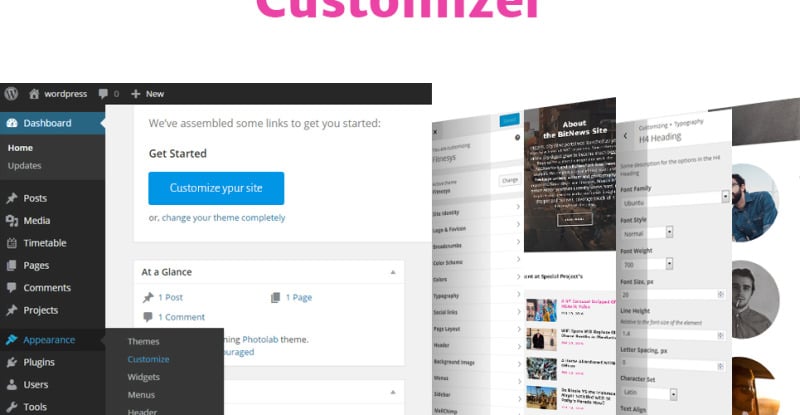The header image appears to be a partially cut-off graphic with the word "Customizer" prominently displayed in a bold, sans-serif font of dark pink or magenta color against a white background. Various screen captures are overlaid in a dynamic 3D arrangement, resembling the interface of a WordPress console. The images depict different types of websites, each partially turned and layered, giving the impression of a rotating gallery of website snapshots.

The most prominent image on the left side is the WordPress dashboard. This dashboard is standard in design, with a primary heading "Dashboard" and a welcome message that reads, "We've assembled some links to get you started." A large blue button labeled "Customize your site" is visible, though "your" is misspelled as "ypur." Below this, there's an option to "change the theme completely."

Additionally, there's a section titled "At a Glance," summarizing the website's status with statistics like "1 Post," "1 Page," and "1 Comment." The WordPress side menu is expanded to the "Appearance" section, and the submenu items including "Themes," "Customize," "Widgets," "Menus," and "Header" are partially obscuring other elements of the dashboard.